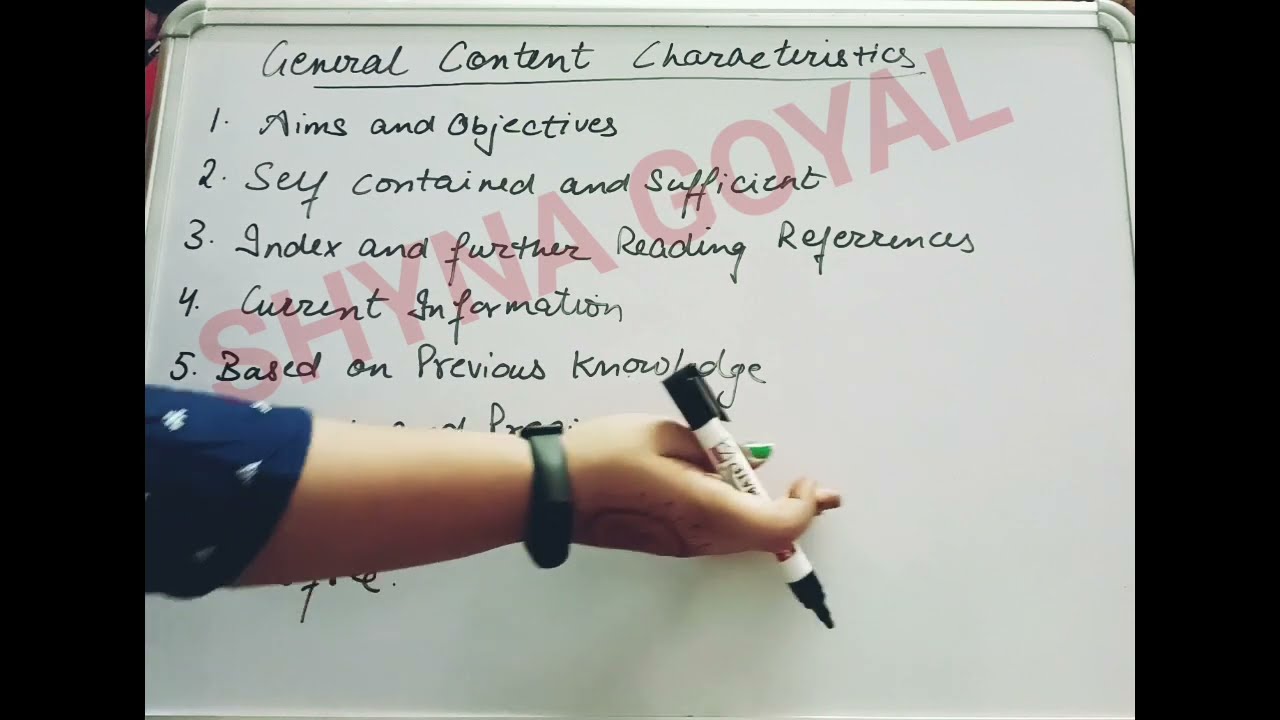The photograph depicts a woman's hand writing on a whiteboard with a black marker. The whiteboard, bordered vertically with black rectangles, features the heading "General Content Characteristics" written in cursive at the top, underlined. Below the heading, a list is visible, numbered one through five down the left-hand side. The listed points include 1) "Aims and Objectives," 2) "SCY Contained and Sufficient," 3) "Index and Further Reading References," 4) "Current Information," and 5) "Based on Previous Knowledge." The woman's arm, which partially obscures more of the list, is light brown or possibly Caucasian, clad in a blue shirt decorated with white cactus patterns, with a black watch strap on her wrist. Her nails are painted green. Covering the image diagonally from the lower left to the upper right is a red watermark reading "SHYNA GOYAL."